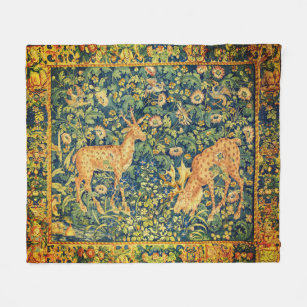The image depicts a medieval-style cloth tapestry adorned with intricate details and rich color. It features two spotted deer-like animals, possibly gazelles or impalas, set within a lush forest scene. The animal on the right, distinguishable by its larger antlers, is bent down nibbling on some greenery, while the other stands alert, gazing forward. Both animals are tan with distinct spots, surrounded by an abundance of grass, flowers, and a vibrant blue-green background interspersed with dark blues and pale greens. The tapestry is bordered by a square frame colored in shades of gold, yellow, and green, with a subtle goldish line demarcating the edge. This exquisite piece appears to be placed against a grayish-white background, highlighting its vibrant hues and detailed craftsmanship. There are no other people or items in the image, allowing the serene natural tableau to fully capture the viewer's attention.